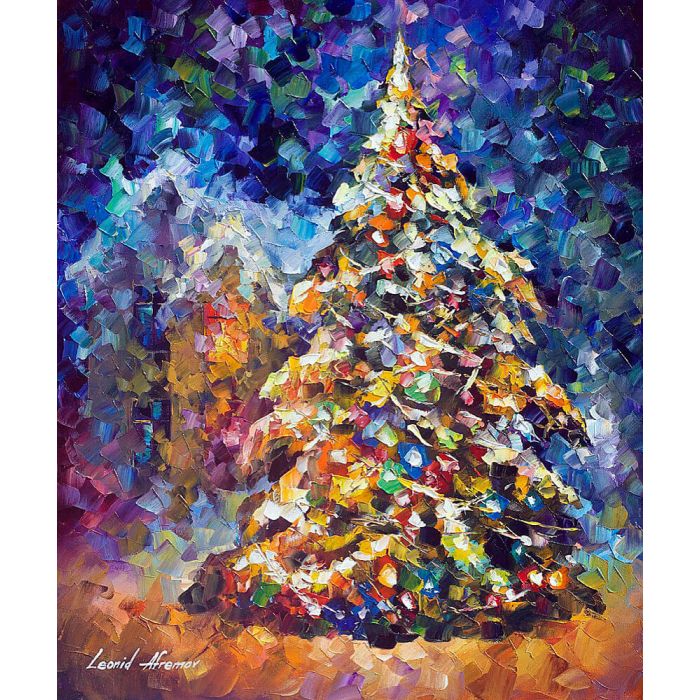This is an abstract, multi-colored painting by Leonid Afremov, signed in white text at the lower left corner. Dominating the vertically rectangular canvas is the artist’s imaginative take on a decorated Christmas tree, composed of vibrant, distinct dabs of paint. The tree, adorned with a myriad of hues including red, blue, and gold ribbons, along with gold bulbs, features a white wreath-like garland and culminates in a white tip. The background transitions smoothly, with the upper left and upper right corners displaying dynamic paint strokes of blue, black, green, and white. The left side blends whites, golds, reds, and yellows, while the right incorporates greens, whites, and grays. Vague human-like shapes can be discerned to the left of the tree, enhancing the abstract nature of the piece. The overall color palette is rich, with purples and blues prominently framing the festive tree in a blend of whimsical brushstrokes.